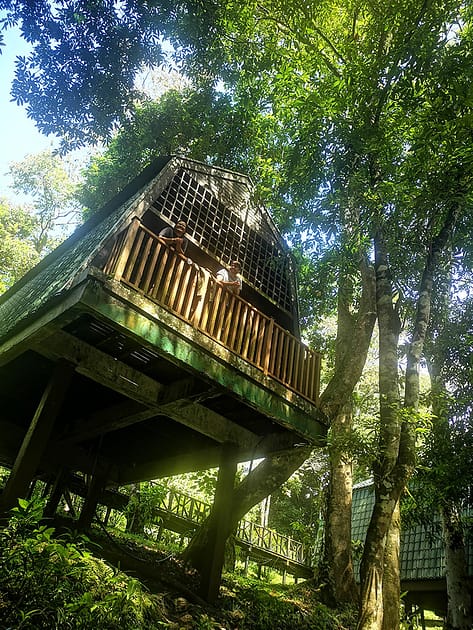The image captures a sunlit outdoor scene featuring a wooden treehouse structure, elevated among leafy green trees. Photographed from the ground looking up, the treehouse is supported by stilts and has a peaked roof with a visible grating and front railing. Two smiling individuals are leaning over the railing, looking down at the photographer. Surrounding the treehouse, additional structures are connected by wooden walkways, hinting at a network of similar platforms. The sunny weather casts light across the greenery, with blue skies and a few white clouds peeking through the leaves. In the foreground, trees with green leaves and brown bark frame the central structure, creating a vibrant and inviting atmosphere.